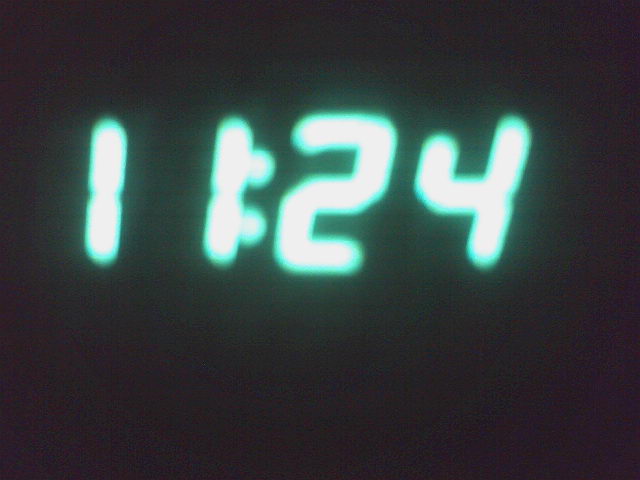A close-up photograph captures the glowing display of a digital clock against a completely black background. The clock shows the time as "11:24". Each digit is presented in a bright white font with a subtle green outline, adding an ethereal glow to the numbers. The "11" is positioned closely together, with the first "1" overlapping the two central dots that serve as the separator. The "2" and "4" following the central dots are also bathed in the same white and green luminescence. The dark surroundings enhance the visibility of the clock's glow, creating a striking contrast between the illuminated digits and the pitch-black background.